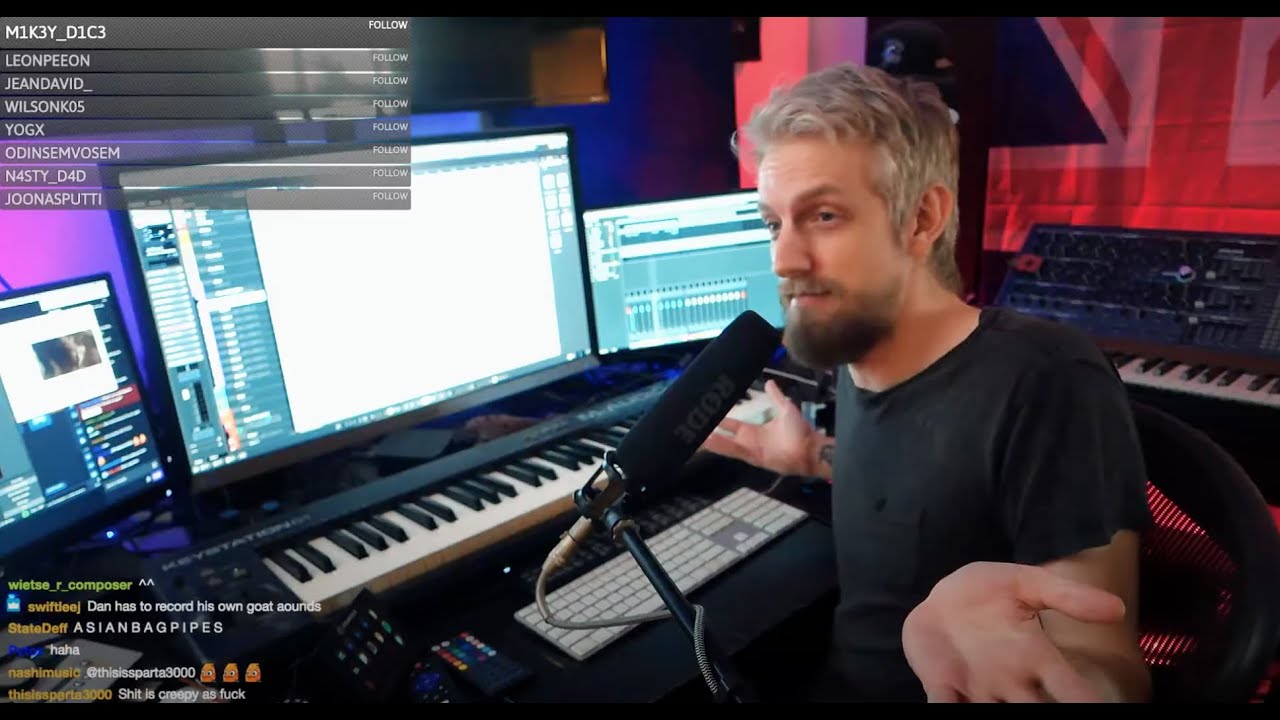Screenshot from a video depicting an engineer in a sound studio. The image features black stripes across the upper and lower edges, likely added by the person who created the screenshot. The engineer is seated in front of two musical keyboards, with a computer keyboard underneath. They are surrounded by multiple monitors, situated to the left, center, and right. Behind them, a synthesizer and a large microphone are visible, poised for use. The engineer's arms are open with their palms showing.

In the upper left-hand corner of the screenshot, various usernames are listed: M1k3y_d1c3 (pronounced "Mikey dice"), follow Leon Peon, follow Jean David, follow Wilson KO5, follow YOGX, follow Odin Sam, follow Vasem, follow Nasty Dad, among others. The bottom left-hand corner contains the text "WITSE are Composer," followed by various possibly garbled phrases such as "swiftly Dan has to record his own goat sounds." Additional dialogue includes a statement about "Asian bagpipes," to which a user humorously responds, "This is Sparta 3000" with chicken emojis. Another user comments, "This is Sparta 3000," followed by a profane remark referring to the content as "creepy."

Overall, the scene captures the high-tech, immersive environment of a sound studio, highlighting both the technical equipment and the casual, humorous interactions between users.